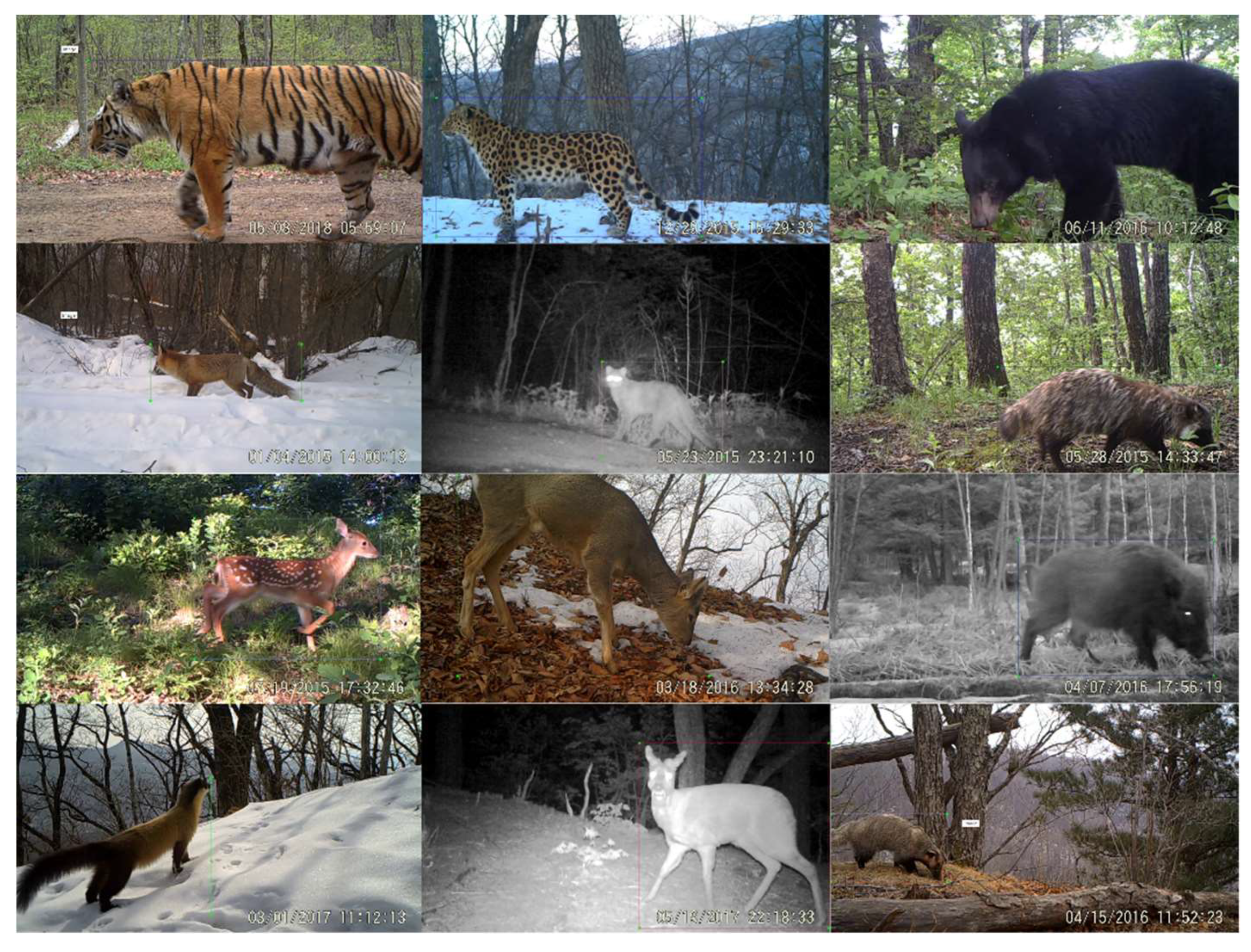This collage consists of twelve trail camera photos capturing a diverse array of wildlife from different natural environments, ranging from reserves and forests to snowy mountainous regions. In the top left, a tiger with its distinctive orange coat and black stripes walks along a dirt path, with a wooden fence visible in the background, suggesting a controlled environment. Next, a spotted cougar roams a snowy mountaintop, followed by a black bear sniffing the ground in a wooded area. The second row begins with a red fox carrying its bushy tail through a snowy landscape, succeeded by a nocturnal, night-vision image of a glowing-eyed mountain lion. A badger with brown fur and white facial markings strides through a forest. A couple of deer occupy the following cells, one a fawn with white spots and the other a doe, both in dense woodland. At night, a wild boar is captured in black and white. On the bottom row, what appears to be a meerkat or tall ferret explores a snowy setting, trailed by another nighttime deer in night-vision, and concluding with another badger. Each image features date and time stamps from 2015 and 2016, underscoring the camera's sporadic operation in varied biomes, regardless of season or time of day.